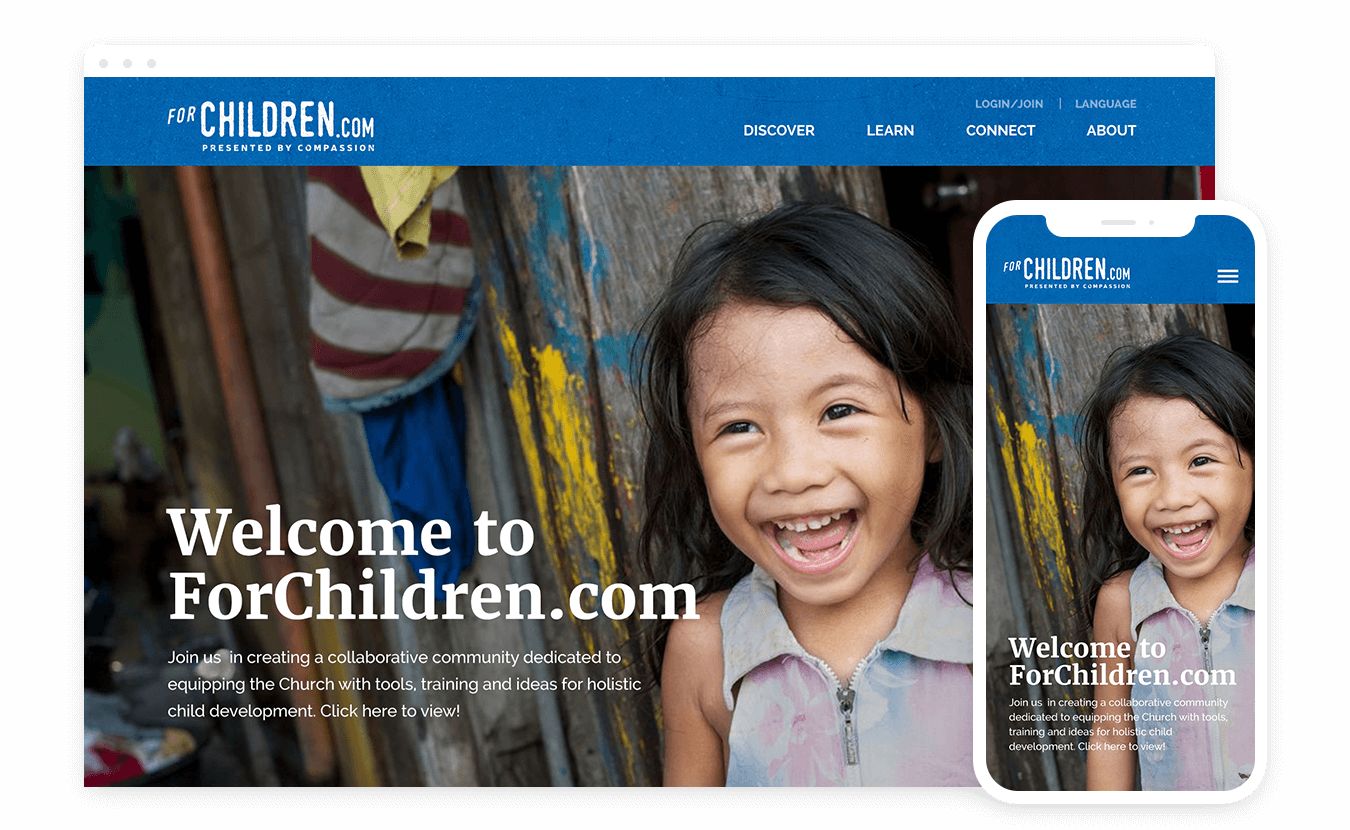In the image, the webpage header features a serene blue background with crisp white text. Positioned at the very top of the page, the header prominently displays "forchildren.com presented by Compassion" on the top-left corner, clearly identifying the site. On the top-right, the header is populated with navigation links including "Discover," "Learn," "Connect," and several others, presented in a clean, readable format. Above these links, there's a language selection option accompanied by an icon resembling a magnifying glass for search functionalities.

The main content of the page hosts a welcoming message on the left side, greeting users with "Welcome to forchildren.com." It invites viewers to join a collaborative community aiming to empower the church with various tools, training programs, and innovative ideas for holistic child development. Accompanying this message is a call-to-action link that prompts visitors to "Click here to view."

On the right side of the main page, there's an illustrative image of a smartphone that showcases what the webpage would look like on a mobile device. The content on the smartphone mirrors that of the main webpage, maintaining consistency in the welcome message and the community invitation. The mobile interface adapts by replacing the navigation tabs with a menu icon – three horizontal lines located at the top-right – allowing users to access the same navigational options ("Discover," "Learn," "Connect") through a collapsible menu. Furthermore, "forchildren.com presented by Compassion" is again displayed at the top-left of the smartphone interface, ensuring brand consistency. The mobile display is completed with a heartwarming picture of a smiling child, adding a personal and emotional touch to the webpage.